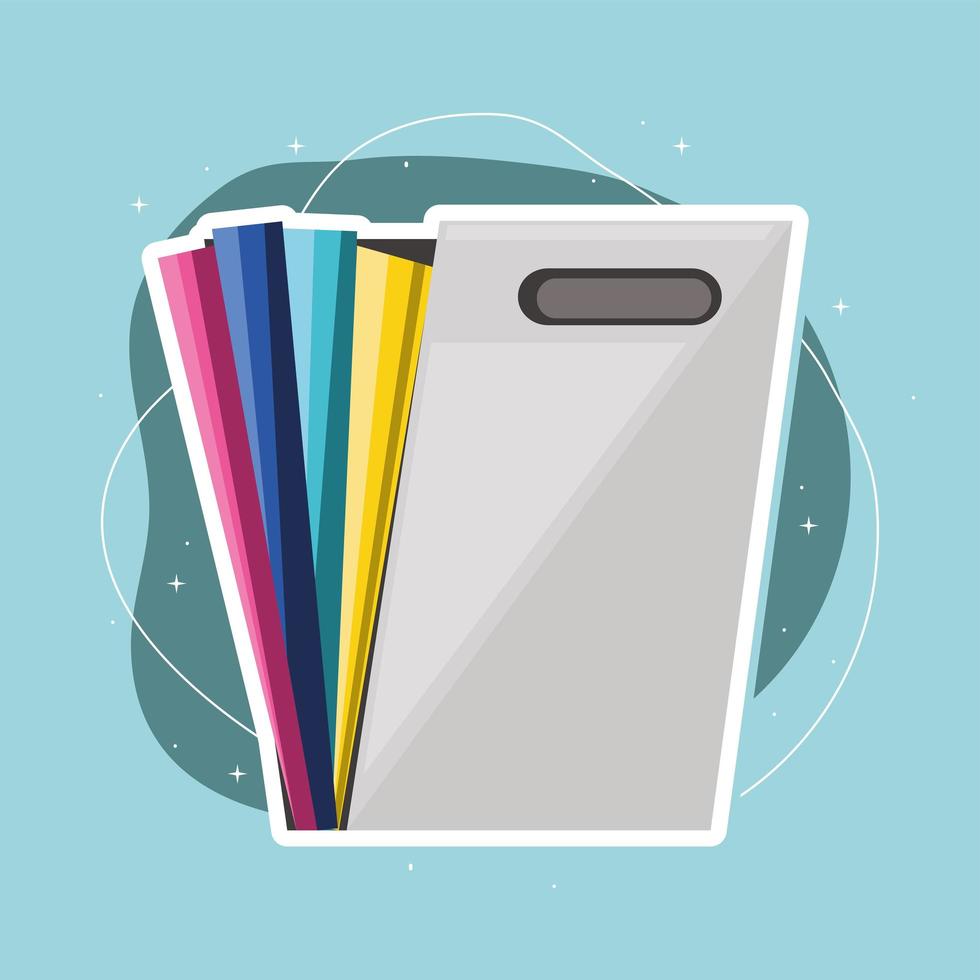This is a highly detailed cartoon illustration of an expandable file folder with a mid-century modern aesthetic. The front of the folder is a light gray color and features an oval-shaped handhold at the top. The folder is opened out, revealing sections with striated colors: pink, blue, light blue, yellow, and purple. These sections show a gradient effect with three variations in each color, such as light pink, hot pink, and dark pink. The colors are wider at the top and gradually narrow towards the bottom, with the pink section remaining the widest. The folder is outlined in white and set against a teal blue background. A dark green, imperfect circle sits behind the folder, and scattered throughout the image are small, twinkling stars enhancing the vintage feel. There is no text or other objects in the image.